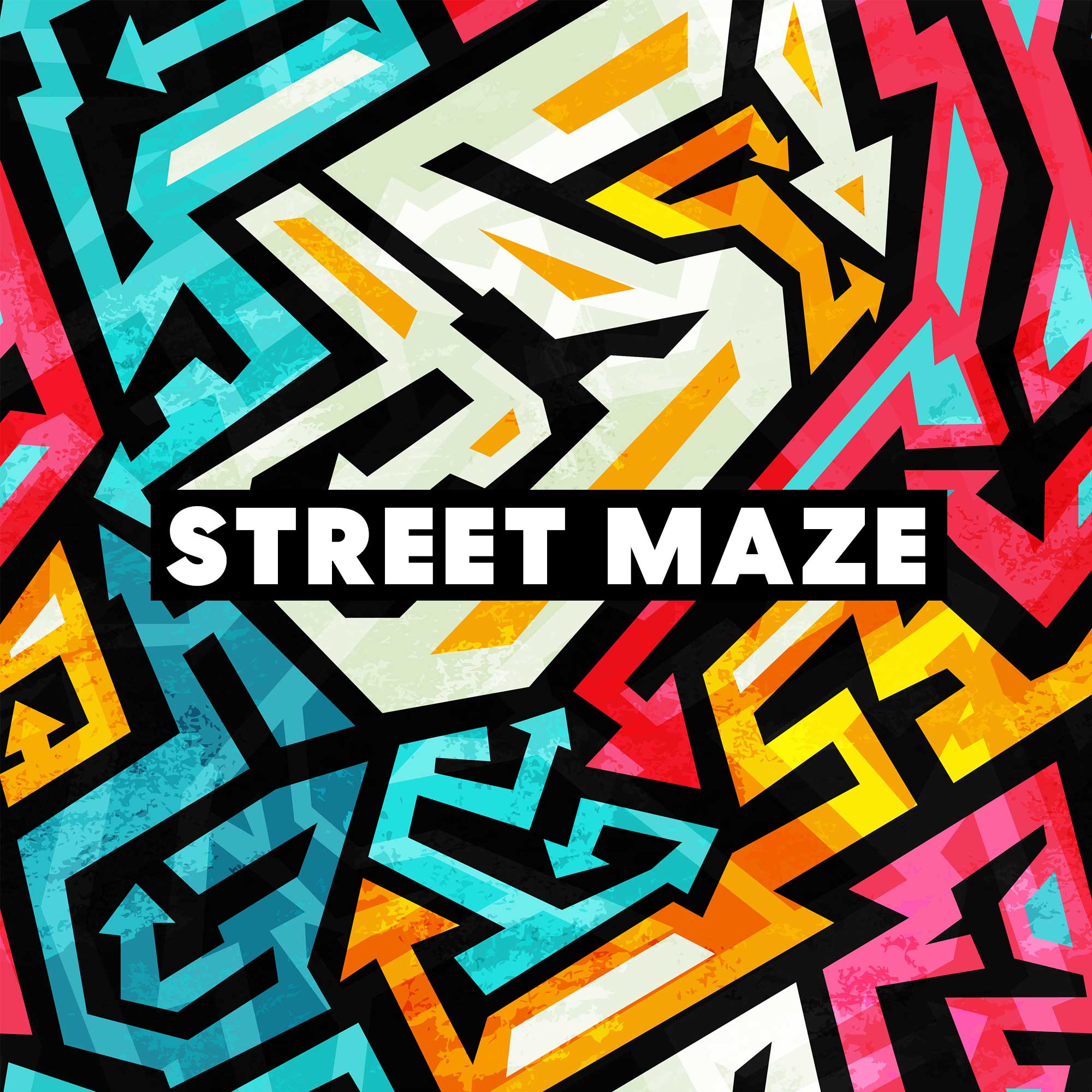The image is a square-shaped, digitally created poster resembling a vibrant and intricate maze. Set against a black background, the maze's boundaries are defined by bright, arrow-like structures in varying hues of yellow, blue, reddish-pink, orange, and gold, with the arrows giving the appearance of graffiti art. Dominating the center of the poster, in bold white capital letters, is the text "Street Maze." The central text is highlighted by a thick black border. This striking combination of colors and patterns, reminiscent of a racing app icon or the start screen of a video game, features no other text or images, focusing attention on the maze-like arrows and the central title.